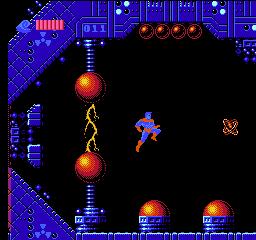A nostalgically-themed screenshot from a retro-style video game. Set against a pitch-black backdrop, the screen bursts with vibrant shades of blue, capturing the essence of classic games from 20-30 years ago. At the center, a cartoonish superhero character, predominantly blue with orange accents, leaps energetically into the air. Surrounding the character are several ominous red spheres, with two of them facing each other, connected by an electrifying arc of yellow lightning. Above, four smaller orbs, blending orange and black hues, are clustered together, while black and white imagery punctuates the top of the screen. To the left, additional smaller blue blocks add to the intricate visual tapestry.